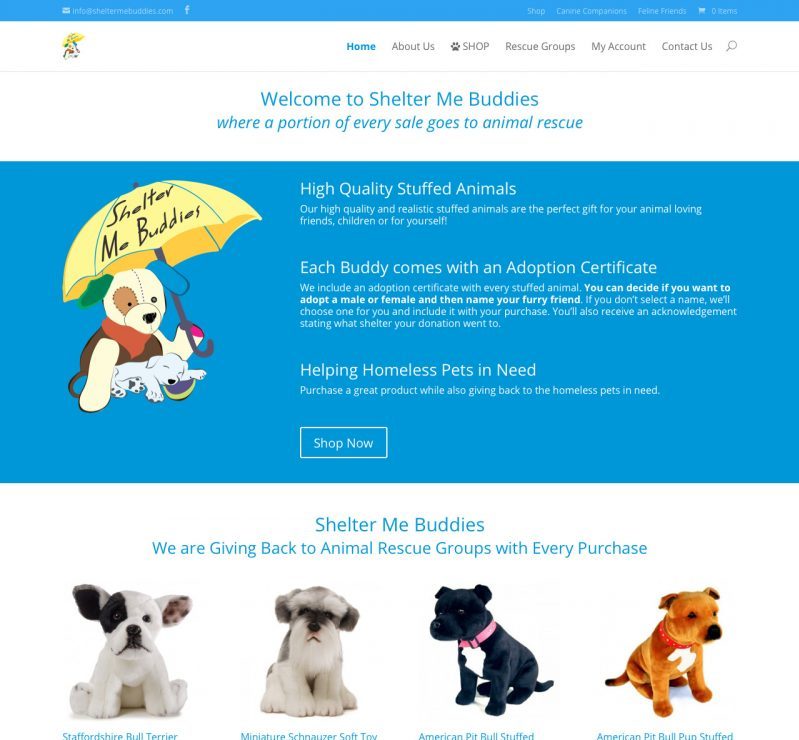This is a screenshot from a shelter's website, adorned with a thin blue border across the top. Positioned on the left side is an email icon that provides the contact email, followed by a Facebook icon. From the right side, there's a display showing "zero items," alongside a white shopping cart icon. The navigation menu includes "Feline Friends," "Canine Companions," and "Shop."

Beneath this header, a white border extends about one-third down the page, featuring a picture of a small stuffed animal dog. The stuffed animal, with a green ear on the left and a blue ear on the right, holds a yellow umbrella that bears the text "Shelter Me Buddies" in black. A small dog is perched across the lap of the stuffed animal. Centrally positioned in blue text, the word "Home" is displayed, followed by "About Us" in black, and then "Shop," "Rescue Groups," "My Account," and "Contact Us." A search icon is located below the "Home." 

In large blue lettering, "Welcome to Shelter Me Buddies" is prominently displayed, followed by the phrase "Where a Portion of Every Sale Goes to Animal Rescue" in smaller blue text. The page transitions to a dark blue background occupying nearly half the view, showcasing the same stuffed animal dog on the right side. The center is dominated by the large text "High Quality Stuffed Animals," with two descriptive lines beneath. Another statement reads, "Each Buddy Comes With an Adoption Certificate," accompanied by a four-line description. Further down, "Helping Homeless Pets in Need" is displayed with a one-line explanation. A blue tab with a white border and the text "Shop Now" in white offers an action prompt. 

Finally, against a white background in the center, "Shelter Me Buddies" is displayed in large blue lettering, with the statement "We are Giving Back to Animal Rescue Groups with Every Purchase" in smaller blue text below. Featured beneath are four stuffed animals: a white one, a hairy dog, a black dog, and a brown dog, each labeled with their names in blue text.